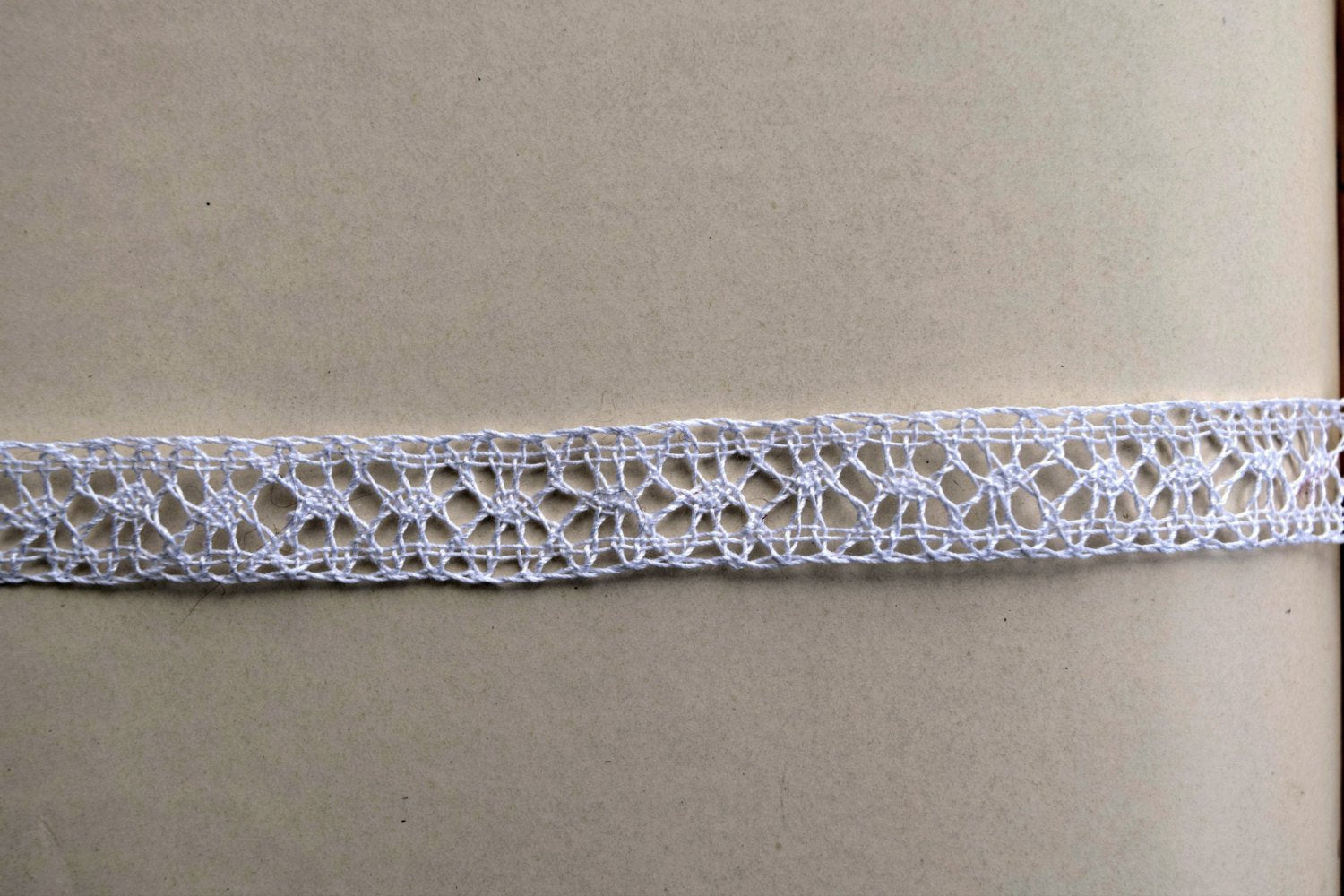The image depicts a long, rectangular piece of lace or tatting, possibly intended as neckwear or a headband, lying on a beige, brownish-tan background speckled with black. The lace, constructed from silver-whitish threads, extends the entire width of the photo. Both the top and bottom edges of the lace are straight and squared off. Along these borders run intricate, web-like patterns with thick centers that resemble circular shapes, from which six or seven stem-like threads extend outwards, creating a design reminiscent of a spider web. The dense lace pattern repeats throughout, allowing glimpses of the background through its large, open spaces.